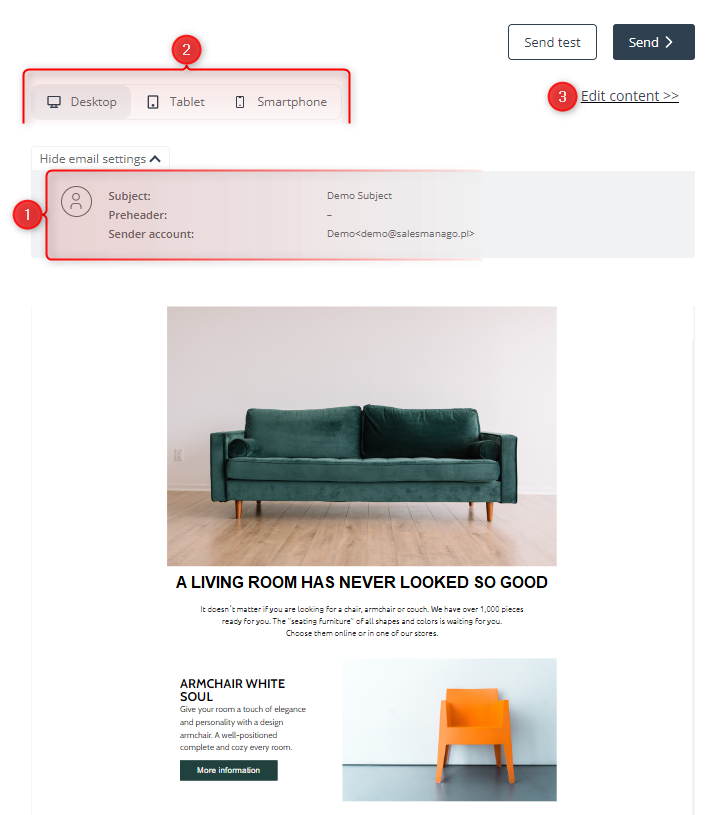The image displays a well-designed web page featuring a vibrant, green leather sofa. The sofa stands out prominently against a pristine white background and is set on sleek wooden flooring. Accompanying the sofa, an orange chair is noticeable in the bottom right corner, adding a pop of contrasting color to the scene.

The web page showcases an alluring caption: “The living room has never looked so good,” emphasizing the visual appeal of the sofa. There are additional textual elements that suggest further descriptive or promotional content about the product. Interactive buttons are present, offering users options for more information or actions related to the sofa.

At the top of the web page, there is a subject line suggesting this might be part of an email advertisement. This email appears to be marked with a pinkish highlight, likely to denote its importance and draw the viewer’s attention to the promotional content. Overall, the web page's layout is clean and aesthetically pleasing, effectively highlighting the sofa and encouraging user engagement.